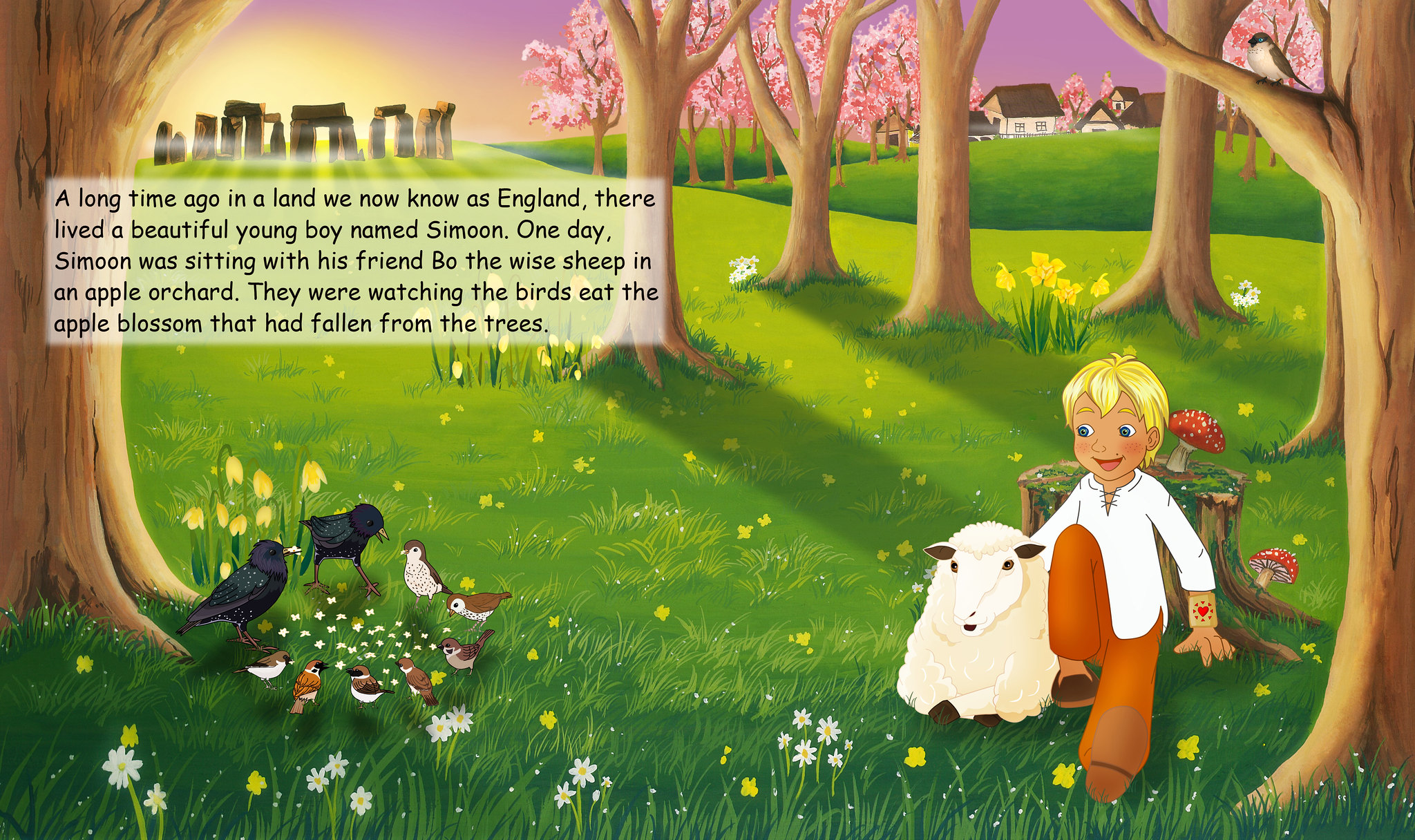The artwork is a detailed fantasy illustration, possibly created by AI, featuring a young boy named Simon. Simon sits against a tree stump adorned with red mushrooms, his tan skin and brown hair standing out against his white long-sleeve shirt, orange pants, and brown shoes. With his arm gently draped over a resting sheep, Simon gazes at a circle of birds on the ground, one of which appears to hold a worm in its beak. The scene is set in a lush forest filled with brown and light brown trees, including cherry blossoms, adding to its magical, Disney-like ambiance. In the background, a residential neighborhood is visible with houses dotting the hilly landscape. The upper left corner of the image features a depiction of Stonehenge bathed in the light of a setting or rising sun, casting a purple hue across the sky. Additionally, a text box narrates the story of Simon and his sheep in a land once known as Scotland. Flowers and weeds, including dandelions, pepper the grass, enhancing the vibrant and whimsical feel of this enchanting scene.